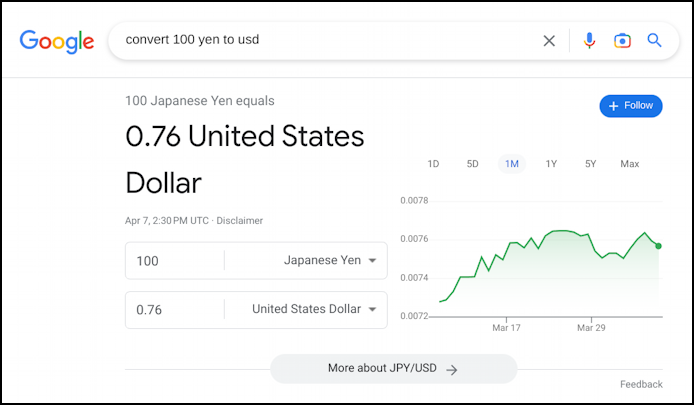The image is a screenshot of a computer screen displaying a currency conversion result in a non-Google Chrome browser. At the top left corner, the word "Google" is depicted in its signature colorful logo. Dominating the top section is an elongated search bar extending across the screen, adorned with an 'X' icon on its right end, followed by a microphone icon, a small square icon, and a search icon. The search query in the bar reads, "convert 100 yen to USD".

Below the search bar, a thin gray line demarcates the header from the main content of the page. Immediately below this line, the conversion result is presented: "100 Japanese yen equals," with "0.76 United States dollars" prominently displayed in bold and larger font beneath it. Further down, there are input fields designed for users to enter different amounts for conversion purposes.

Occupying the right side of the screen is a graphical representation of the currency exchange rate. This graph features a light green, squiggly line indicating fluctuations in the exchange rate over time. The graph provides options to view data ranges from one day to five years, extending to a maximum range. The Y-axis displays decimal numbers to indicate the value scale.

At the very bottom of the screen, a gray button labeled "More about JPY/USD" is accompanied by a right-pointing arrow, indicating additional information is available upon interaction.